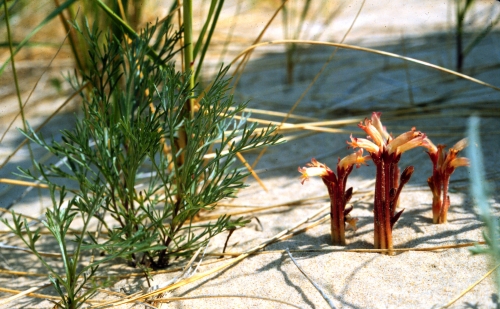An outdoor photograph captures a sandy, sunlit scene that resembles a beach or coastline rather than an underwater environment. The ground is predominantly light tan sand, which is bright in the front and back corners of the image, but shaded in the middle, possibly by a large tree. In the lower right-hand corner, there are intriguing red plants that almost resemble underwater coral, but their presence in this sunny, above-ground scene suggests they might be wildflowers or mushrooms with dark brown stems and tan tops. On the left side, a clump of deep green, tall grass with some yellow-tipped blades is prominently featured. Additionally, various other types of thin green plants and some bamboo-like structures are visible, sprouting from the sandy soil amidst the textured shadows.